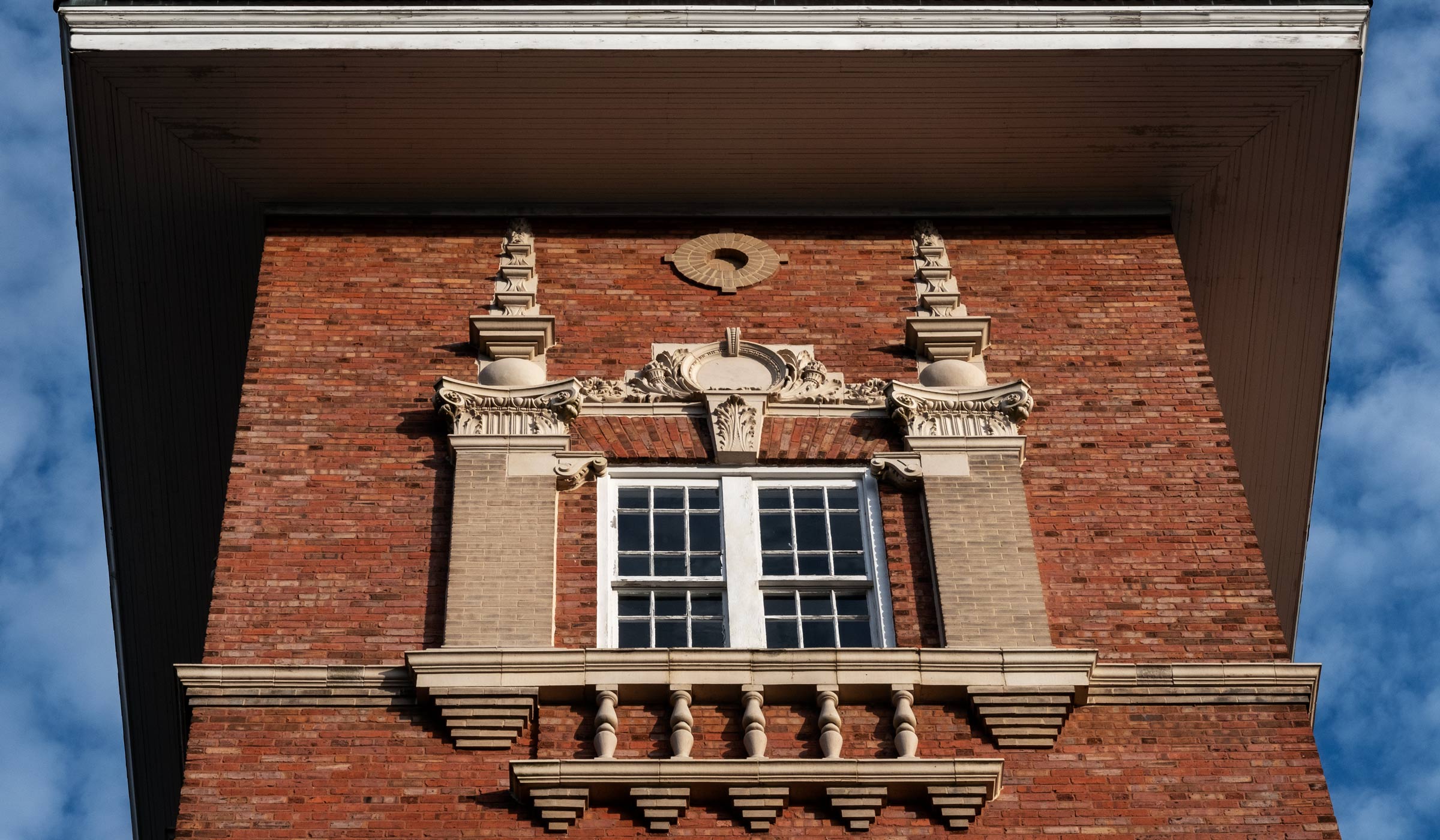In this color photograph, taken at an upward angle, the focus is on the upper part of a historical red brick building adorned with intricate architectural details. The center of the image showcases a large white window with a small false balcony and ornate scroll work below it. This window is framed by pillars featuring detailed decorations. Above the scroll work lies a round metal shape set against the brick façade. The rooftop, which extends wider than the building itself, is a dark brown material with white trimming. The background of the photograph captures a deep, slightly moody blue sky filled with fluffy, overcast white clouds on both the left and right sides. The overall scene is devoid of people and any visible text, highlighting the building's striking details against the dynamic sky.